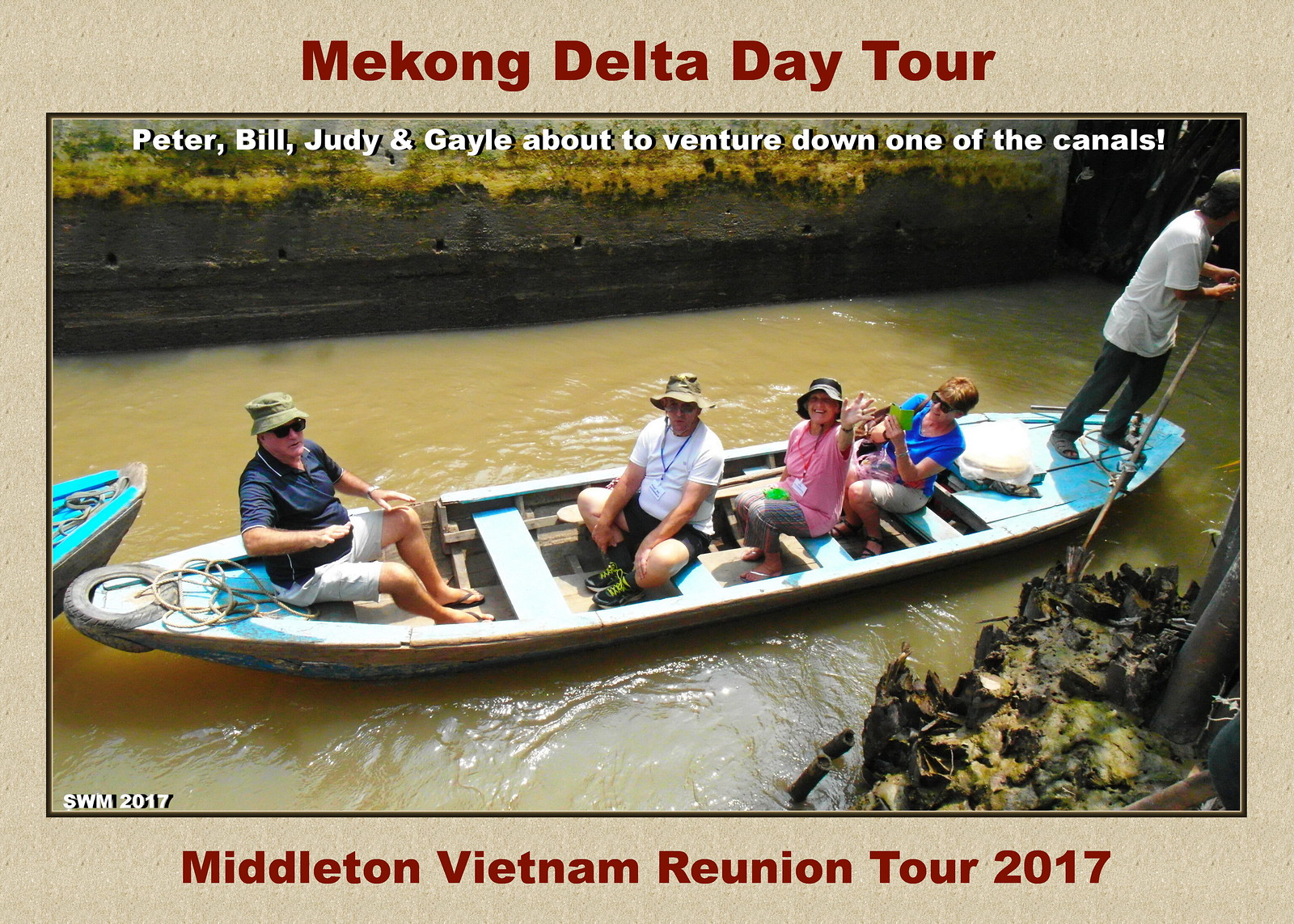This color photograph captures a serene moment during the "Mekong Delta Day Tour," as indicated by the bold red print on the beige border framing the image. Four white American tourists—Peter, Bill, Judy, and Gail—are seated in a long, canoe-like boat navigating the brown waters of a Mekong Delta canal. At the rear of the boat, a local Vietnamese man stands, skillfully steering with a long pole, reminiscent of an Italian gondolier. The backdrop features a retaining wall, emphasizing the canal setting. The caption further identifies the scene as part of the "Middleton Vietnam Reunion Tour 2017," marking a memorable adventure for the group.